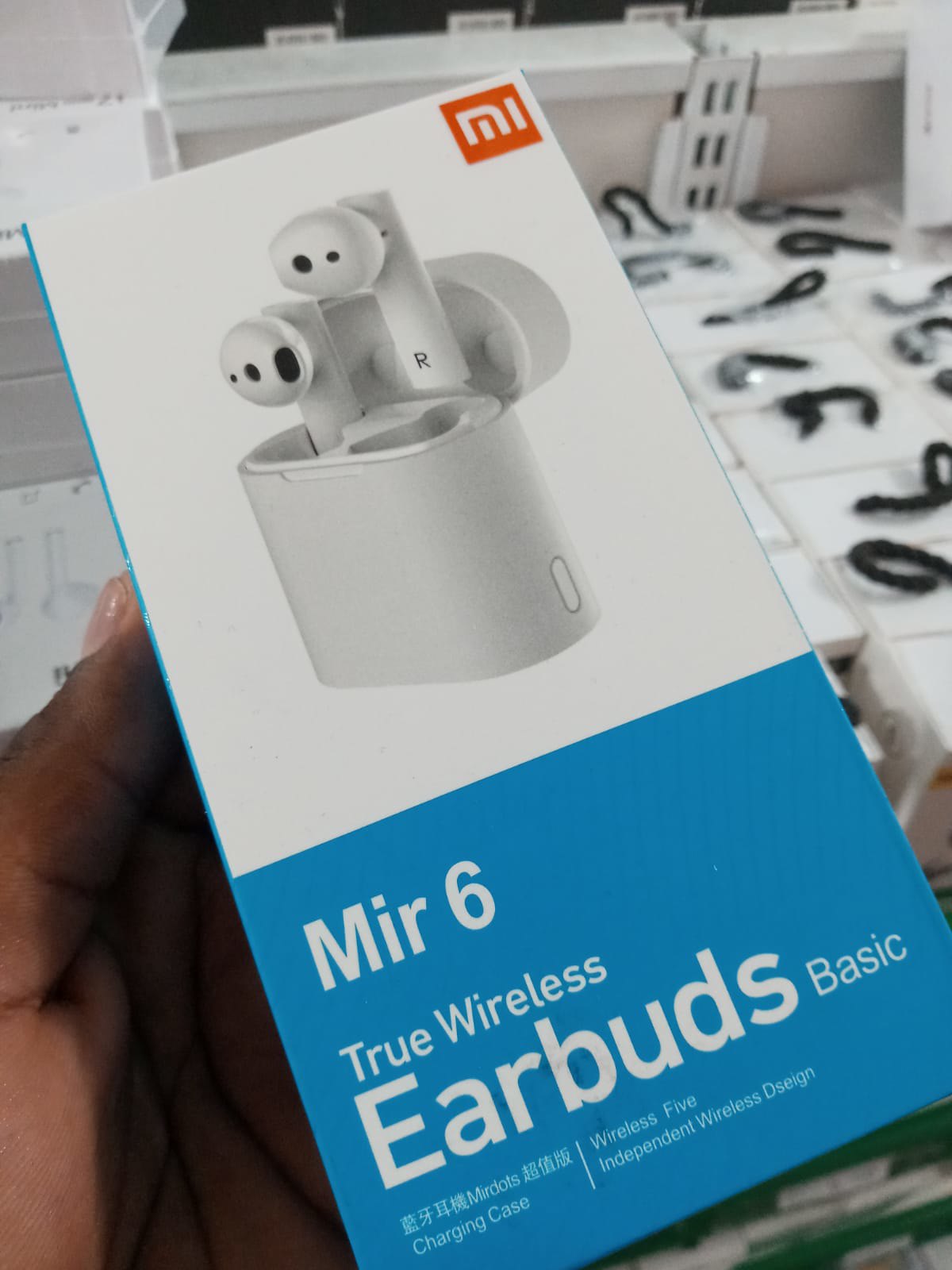This indoor color photograph features a close-up view of a new box of earbuds held in a left hand, which extends from the lower left corner of the image. The hand is partially visible, showing the thumb. The box itself is visually divided into two sections: the upper two-thirds, which has a white background displaying the earbuds and their carrying case in a three-quarter view, and the lower third, which has a light blue background with white lettering that reads, "MIR6 True Wireless Earbuds Basic."

The depicted earbuds are white, with one partially seated in the open white case and the other lifted out, showing an "R" engraved on its stem, indicating the right earbud. The image is relatively dimly lit but in focus, capturing fine details like the "Charging Case" and "Wireless 5 Independent Wireless Design" text on the box, as well as some foreign characters and the word "MIRDOTS."

The background is slightly out of focus, featuring what appear to be numbers on a calendar shaped from black materials like straw or pipe cleaners. Additionally, some fabric straps lining a white table are discernible, and the overall setting seems to be a shop, given the white-topped boxes with dark handles seen behind the hand, suggesting items for sale.